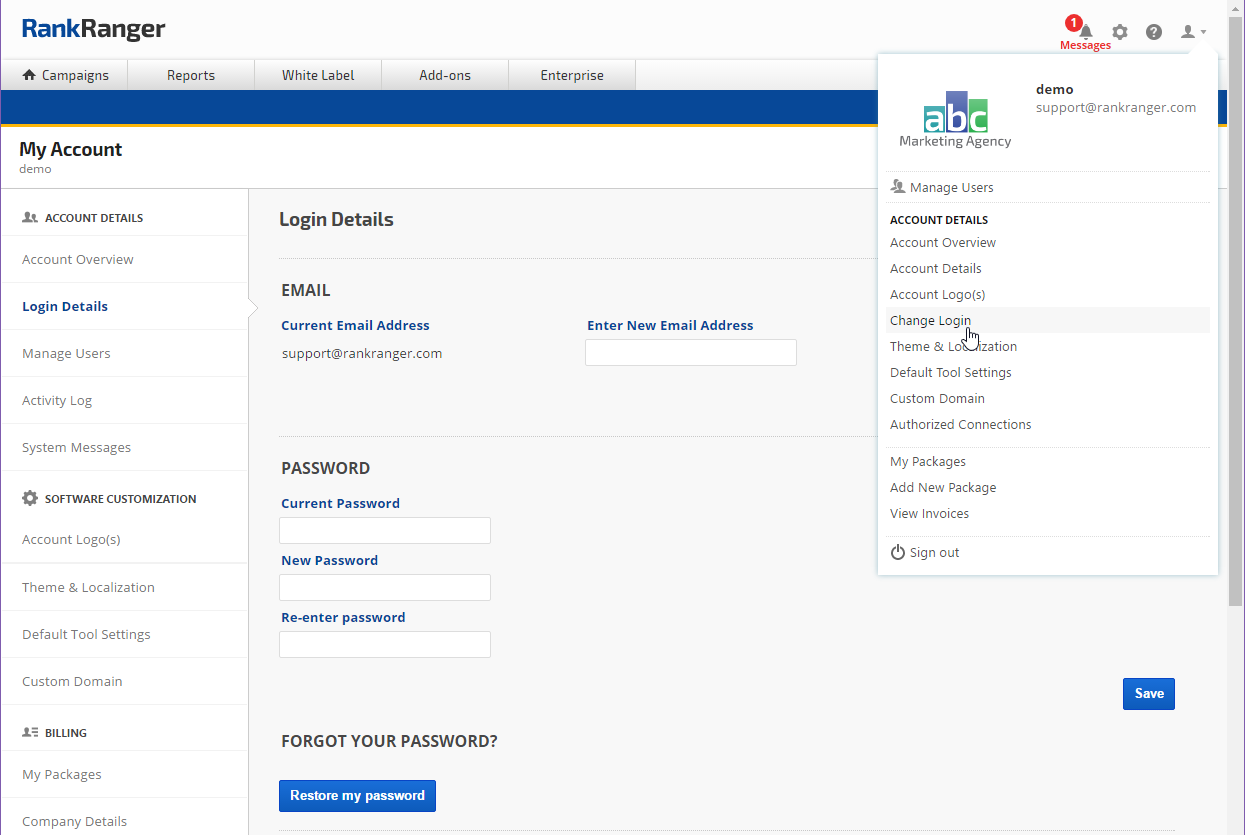The image predominantly features a light blue background. On the right side, there is a slightly darker blue section. At the top, a light blue box labeled "Rank Ranger" is visible, with "Rank" in blue and "Ranger" in black. A bell icon with a red circle indicating one notification, a red "Messages" icon, and a dropdown menu in a white box outlined in blue are also present. The dropdown includes "ABC Marketing Agency" in white letters inside teal and green boxes, "demo@support.RankRanger.com," sections for managing users and account details, and a blue "Change Location" button with a pointer on it, followed by a "Sign Out" option. 

On the left side, there is a section labeled "My Account Demo," followed by a vertical line. Below is a white background containing several boxes. The first box has "Account Details," followed by "Login Details," "Software Customization," and "Billing." The right side of the image prominently features a large blue box labeled "Login Details." Beneath this is a line and sections for "Email," showing the current email address "support@RankRanger.com" in blue and a field to enter a new email address in blue with a white input box. Further down, there are sections for "Password," including "Current Password" in blue with a white input box, "New Password" in blue with a white input box, and "Re-enter Password" in blue with a white input box. A "Forgot Your Password?" option in black text is followed by a blue button with "Restore My Password" in white text. On the far right, there is a small blue button labeled "Save" in white text.